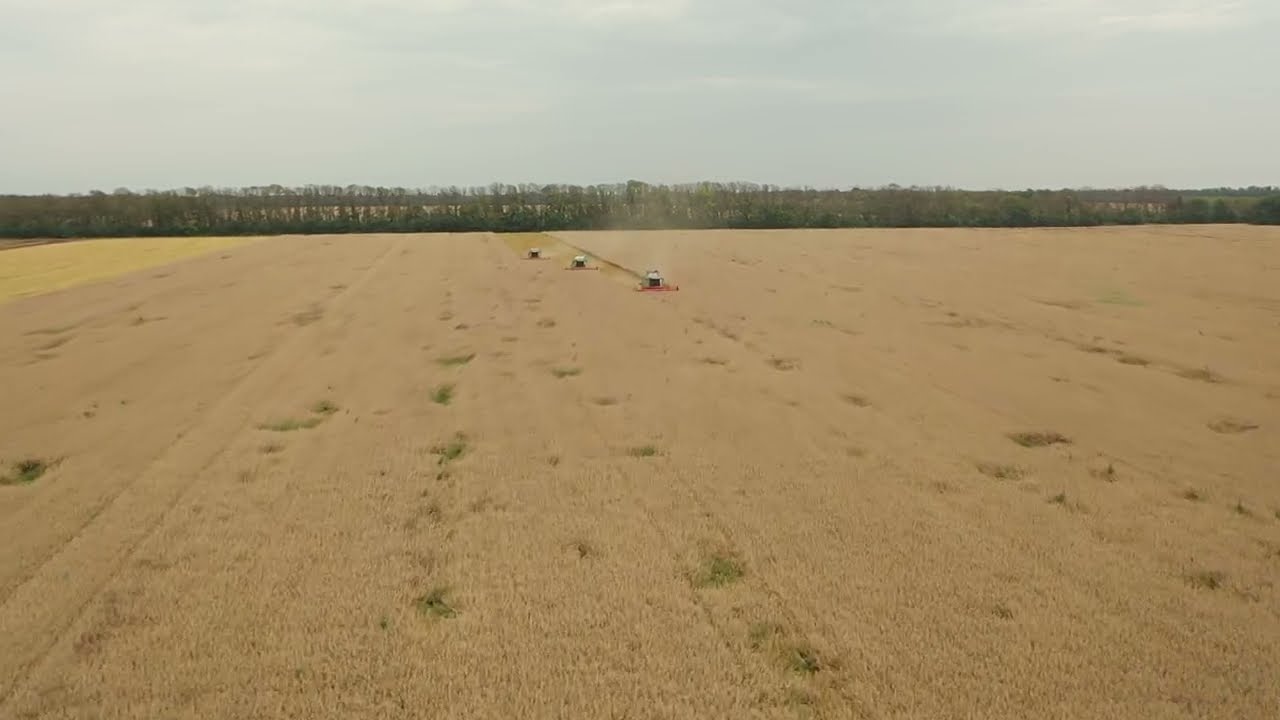An aerial view captures a sprawling farm field being harvested by three distinct tractors in the center. The tractors move in a pattern that angles slightly to the left, plowing through golden plants that resemble wheat. The closest tractor, on the right, features a red front and a green body. The center tractor also boasts a red front and green body, while the leftmost one is yellow with a red front. The field, covering the bottom half of the image, is mostly flat, dotted with patches of short green growth amidst the dry, trimmed grass. A tranquil yet industrial agricultural scene unfolds under a dark gray, overcast sky with scattered white clouds. On the horizon, a row of leafless deciduous trees stretches across, hinting at a season of fall or early spring. Peeking through the trees, another farm field can be glimpsed, enhancing the sense of vast, cultivated land.